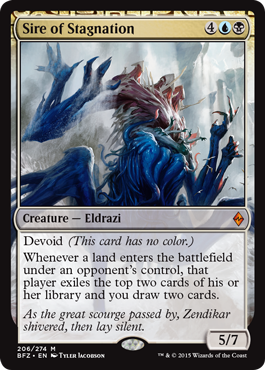The image depicts a Magic: The Gathering trading card titled "Sire of Stagnation." The card's name is prominently displayed at the top in red text, set against a yellowish-gold border. To the right of the name are three circular symbols: the first contains the number four, the second a raindrop, and the third a skull. The illustration on the card features a monstrous creature with a blue lower body and a red upper body, surrounded by floating islands. Below the illustration, the card designates the creature type as "Eldrazi" in white text beside an orange triangle. Just underneath, the text "Devoid" signifies that the card has no color. Further down, an ability description reads: "Whenever a land enters the battlefield under an opponent's control, that player exiles the top two cards of their library and draws two cards."